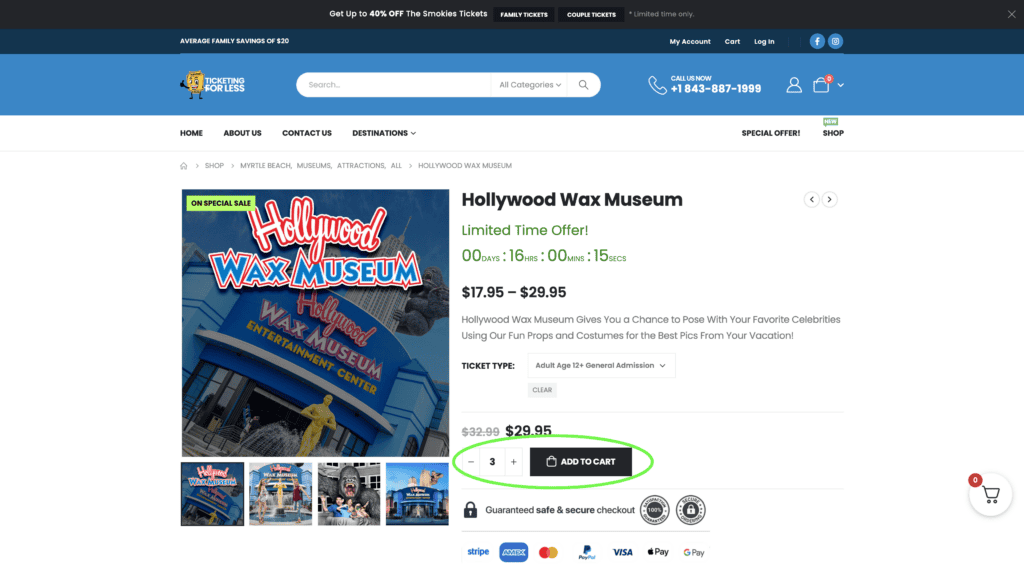This image is a detailed screenshot of the "Ticketing for Less" website, captured from a desktop view. The webpage has a predominantly white background with a blue banner at the top featuring a cartoon yellow ticket character giving a thumbs up. The text "Ticketing for Less" is displayed in white on the blue banner, located next to the ticket mascot.

In the upper left corner, there's a search box with a dropdown menu for categories, and adjacent to it, contact information and various interactive icons are visible. Below the banner, a navigation header includes clickable links for "Home," "About Us," "Contact Us," and "Destinations," along with dropdown menu options.

The main content area prominently features a special offer for the Hollywood Wax Museum. A timer indicates there are 16 hours and 15 seconds left in the limited time offer, with ticket prices ranging from $17.95 to $29.95. Descriptive text highlights the opportunity to pose with favorite celebrities at the museum. Accompanying the description are multiple images of the Hollywood Wax Museum. A green outline highlights the "Add to Cart" button, indicating that three tickets have already been added to the shopping cart.